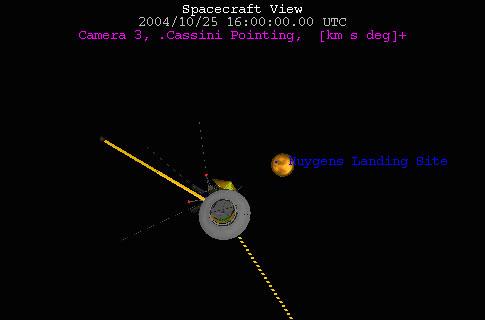The image is a low-quality space photograph with a completely black backdrop. At the top in white lettering, it reads "Spacecraft View," followed by the date "2004-10-25" and the timestamp "16:00:00.00 UTC." Below this, in purple lettering, it says "Camera 3, Cassini Pointing, (KM S DEG)+." The right-hand corner features blue lettering that reads "Huygens Landing Site." The central elements of the photo include a gray satellite-like object and a bright yellow orb labeled as "Phrygian's landing site." Several lines overlay the image: a solid yellow line extends diagonally upward from near the satellite, a yellow dotted line descends from the bottom of the satellite, and two vague white dotted lines are also present.